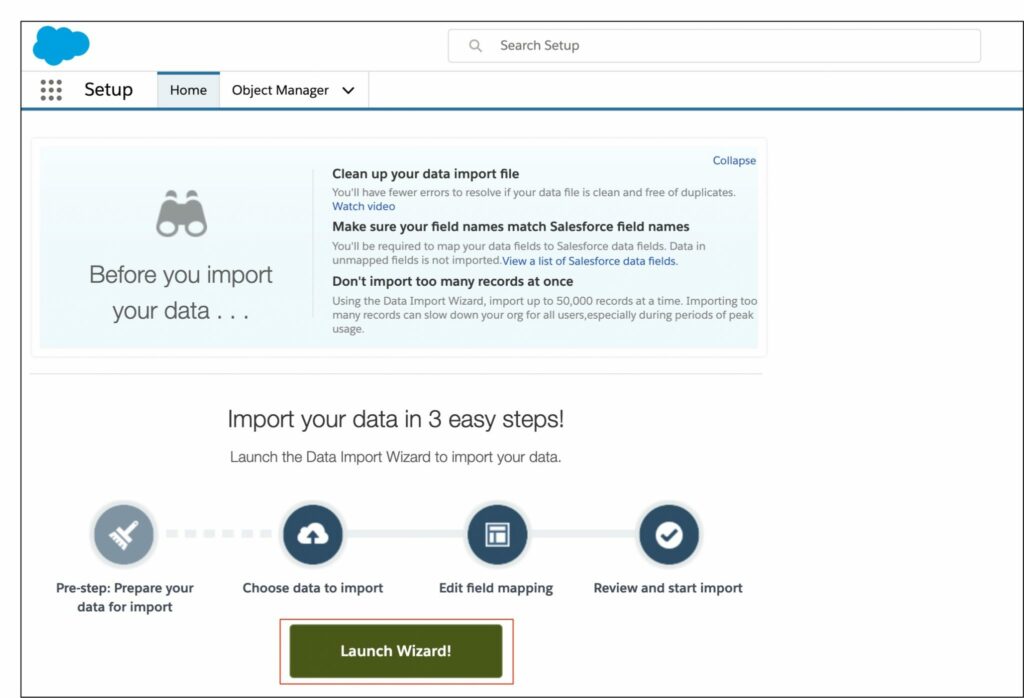Here’s your revised and detailed caption:

The image depicts a software interface, likely an installer or setup wizard, displayed on a computer screen. In the upper left-hand corner, there is a blue cloud motif, indicative of a cloud-based service. The upper right-hand corner features a long search bar equipped with a magnifying glass icon, designed for search functionality.

Below the search bar is a navigation taskbar with tabs labeled "Setup," "Home," and "Object Manager." A blue divider line separates these from the main content area. Positioned on the left-hand side, there is a light blue information square with binoculars and the text "Before you import your data..."

On the right-hand side, detailed instructions are provided:

1. **Clean Up Your Data Import File:**
   - Ensuring the data file is clean and free of duplicates will reduce errors during import.
   - A link labeled "Watch Video" offers further guidance.

2. **Field Name Matching:**
   - It's crucial to match your field names with Salesforce field names, as unmapped fields won't be imported.
   - A link labeled "View a list of Salesforce data fields" provides a reference for field names.

3. **Importing Records:**
   - It’s advised not to import too many records at once. The wizard supports importing up to 50,000 records to avoid slowing down the organization, especially during peak usage.
   - This section can be collapsed for convenience.

At the bottom, step-by-step directions include "Preset," "Choose Data Import," "Edit Field Mapping," "Review," and "Start Import." A prominent green button with red-highlighted corners is labeled "Launch Wizard."

The entire interface is set against a clean white background, contributing to a user-friendly and organized layout.